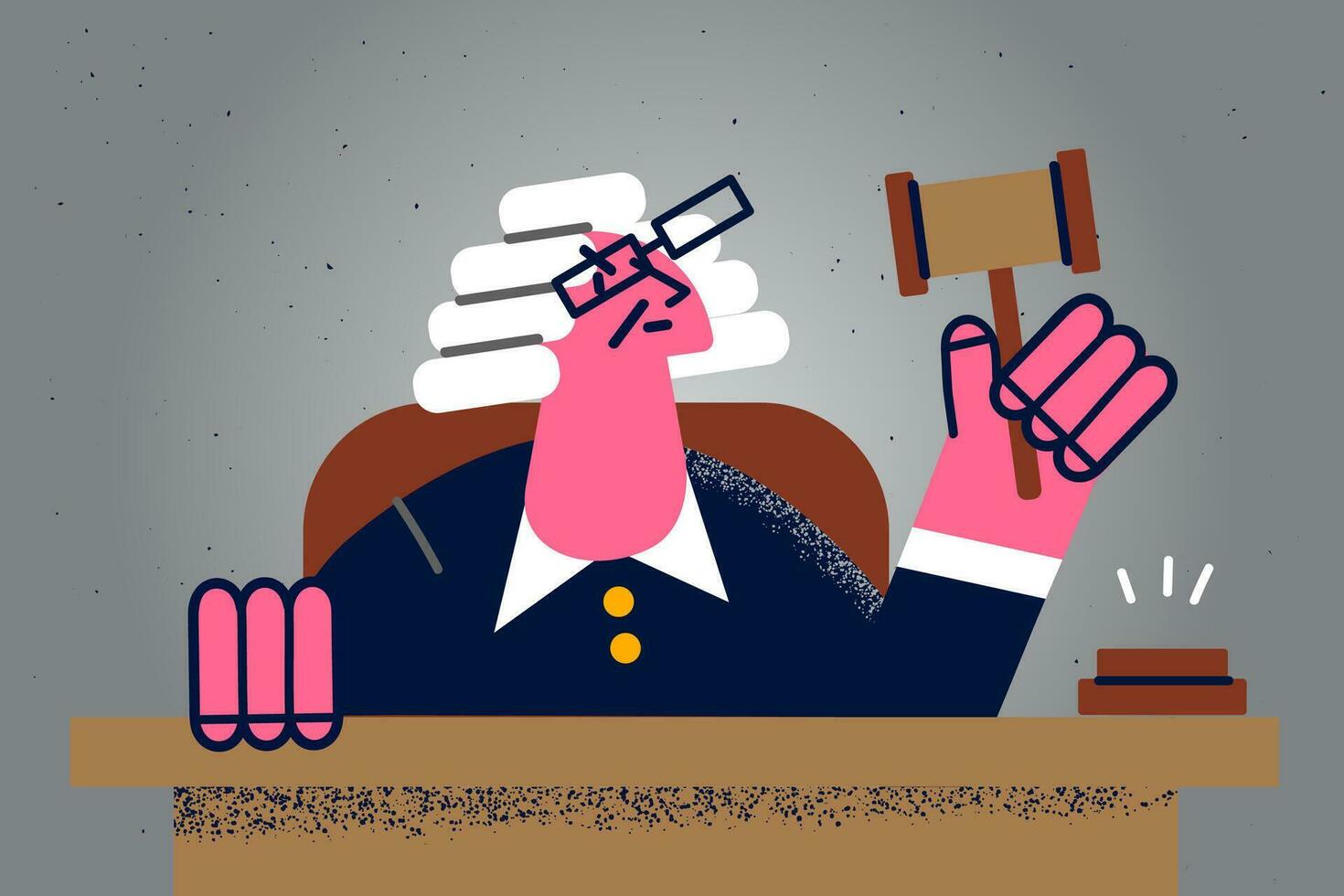The image portrays a cartoonish and minimalistic depiction of a judge, likely computer-generated, with a blocky style. The judge is characterized by a bold use of colors and outlines, featuring distinct and exaggerated elements. He has coral pink skin, accentuated by white hair, and is wearing a traditional 18th or 19th-century powdered wig. The judge's robe is a dark navy black, adorned with two yellow buttons and a white collar. 

Seated behind a tan desk with darker shadows delineating its structure, the judge holds a gavel in his large left hand. The gavel appears recently struck, indicated by three white lines above its seat, suggesting a noise or impact. The force of the strike has caused the judge's glasses to become askew. The background is a darker gray color, while the judge's chair is brown. Overall, the image combines minimalistic and cartoonish aesthetics, reminiscent of the style of Peppa Pig but applied to a human judge, emphasizing bold outlines and vibrant colors against a subdued background.